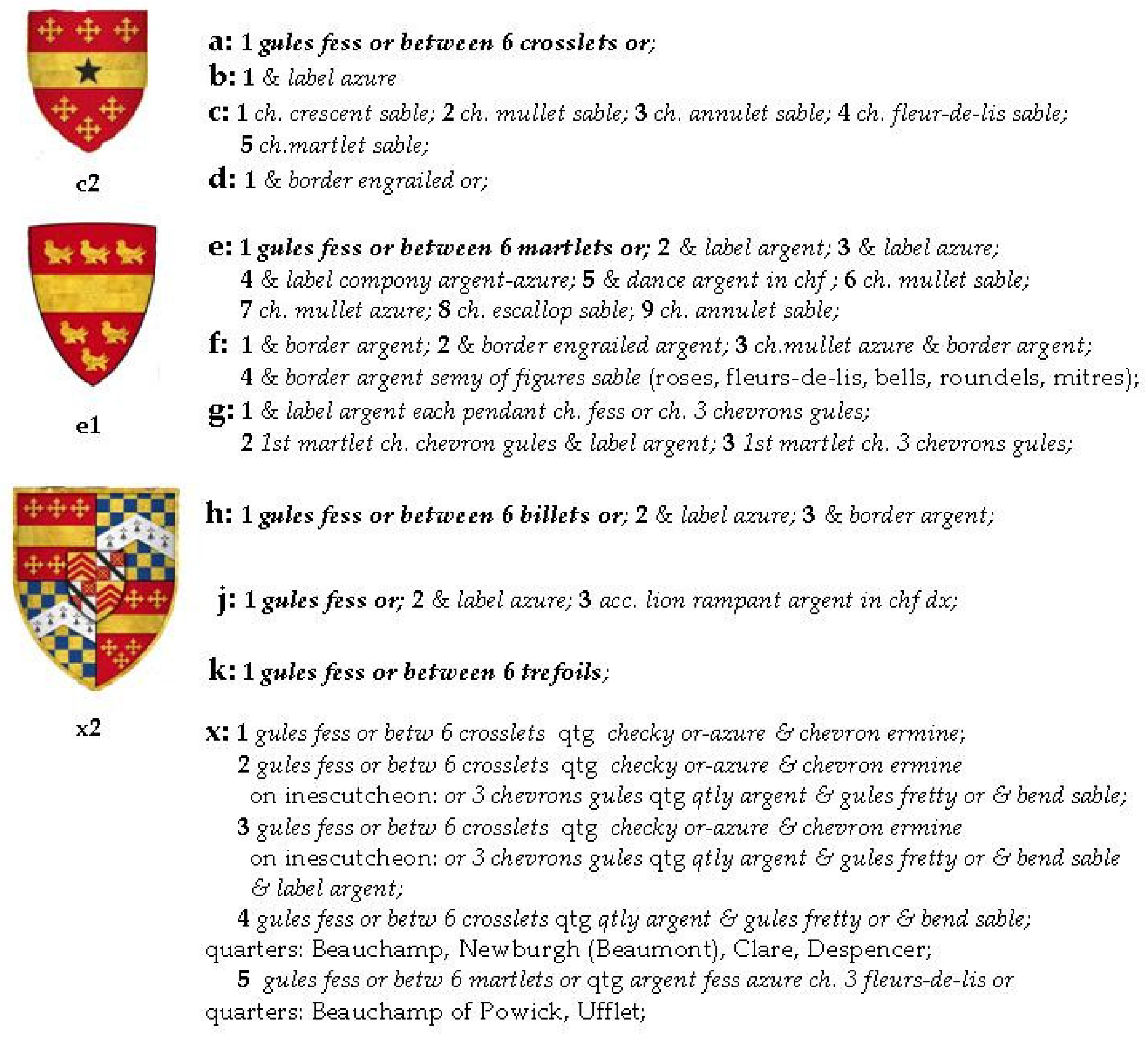This image features three distinct coat of arms or crests aligned vertically on the left side against a plain white background. The crests exhibit intricate designs in red, gold, black, blue, and green, accompanied by detailed textual descriptions on the right side.

The first crest at the top includes red and gold colors with three gold crosses on a red field, a gold band with a black star, and a triangular section with three more gold crosses. This crest is labeled as C2.

The second, taller crest predominantly features a burgundy background adorned with gold elements. At the top, there are three gold birds, followed by a gold stripe in the middle, and three additional gold birds at the bottom. It is labeled as E1.

The third crest, equally proportioned in height and width, has a complex design with blue and gold checkers in the upper right and lower left corners. A white banner with black symbols in an upside-down V shape spans across, along with sections of gold and red crosses, arranged in an alternating pattern. This busy crest is labeled X2.

To the right of the crests is a detailed ledger listing various elements denoted by letters A through J and X, followed by semicolons and numerals, explaining the symbolic features of each coat of arms. The color scheme, the symmetrical placement of symbols, and the precise illustrative style highlight the heraldic significance of the crests, with all written information displayed in black text on the white background.